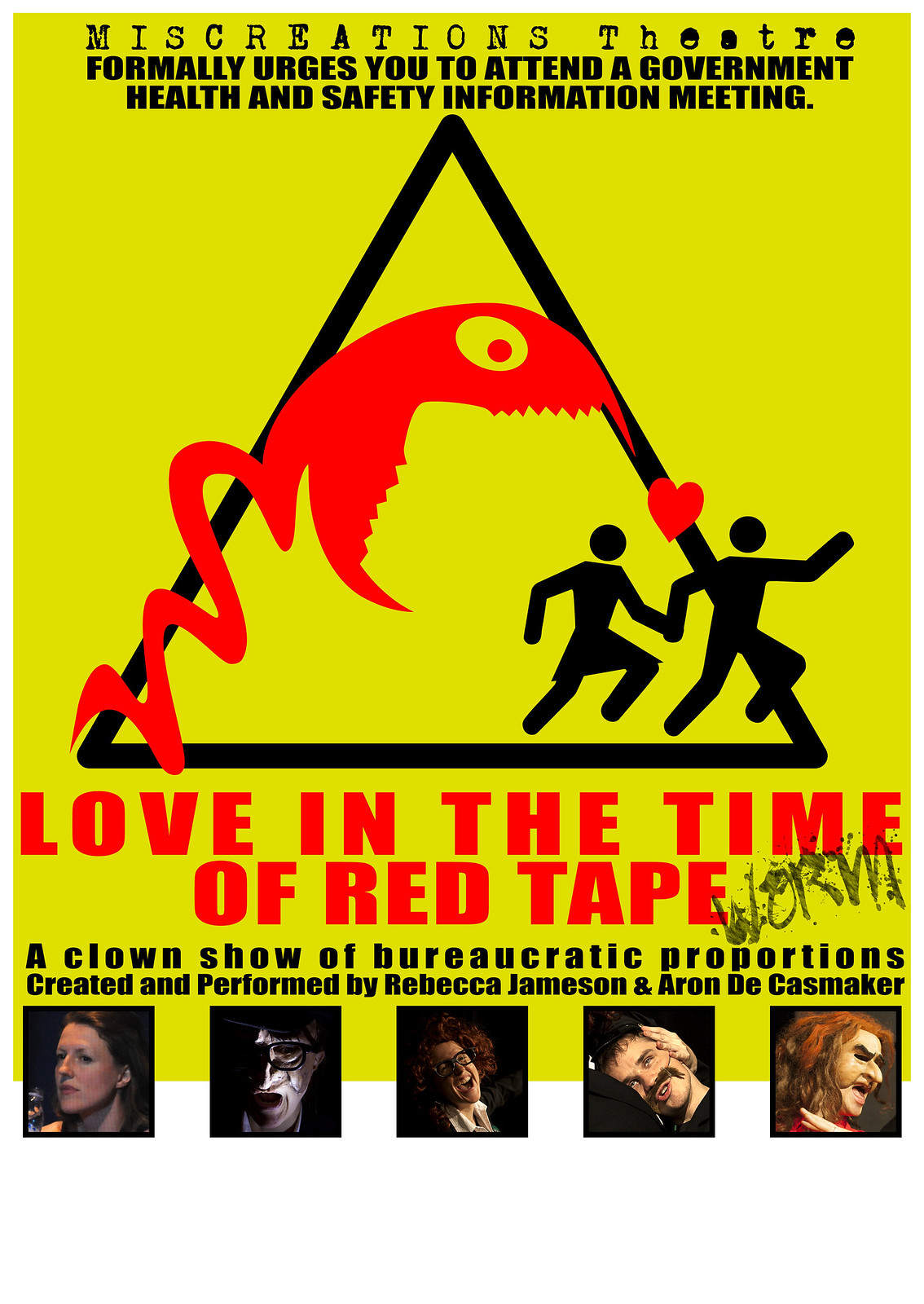The poster, set against a vibrant yellow background, advertises a theater production by Miscreations Theater, entitled "Love in the Time of Red Tape." At the top, black text formally urges attendees to join a government health and safety information meeting. The central artwork features a black triangle framing a surreal scene: a red, worm-like monster with an open mouth and fangs chases two black stick-figure-like individuals, symbolizing a couple with a red heart floating between them. Overlaying the triangle, the title text in red declares "Love in the Time of Red Tape," with "Worm" in graffiti-style font beside it. Below, black text announces, "A Clown Show of Bureaucratic Productions Created and Performed by Rebecca Jameson and Aaron De Kazmaker." Accompanying this are five boxed images of the performers: from left to right, a woman, a man in a silver mask, a laughing man with curly red hair and glasses, a man with a large mustache leaning on someone’s lap, and a person with witch-like makeup and red stringy hair.